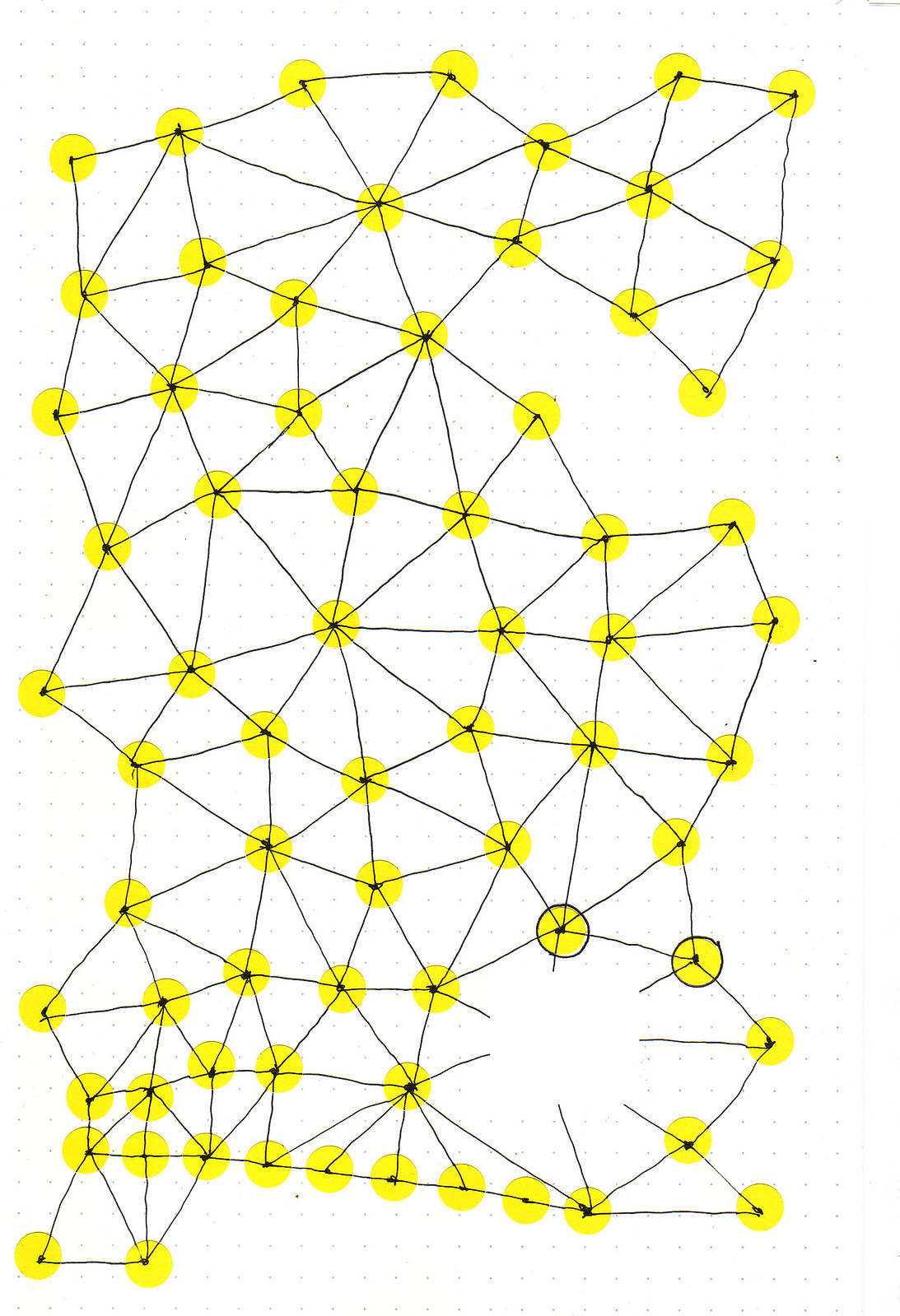The image features numerous yellow circles interconnected by black lines. The black lines converge at the centers of the yellow circles, forming a complex network. Predominantly, these lines create triangular formations, with each triangle having one circle at its apex and two at its base. This pattern of triangular shapes is consistent throughout the image.

However, as you move toward the bottom of the image, these shapes begin to vary, with some triangles transforming into right-angled triangles and other geometric forms. Additionally, the arrangement of the yellow circles at the bottom becomes denser and more tightly packed, with approximately nine circles closely clustered together. This contrasts with the more sparsely spaced triangles seen in the upper portions of the image. The network of black lines remains consistent, emanating from the centers of all yellow circles.